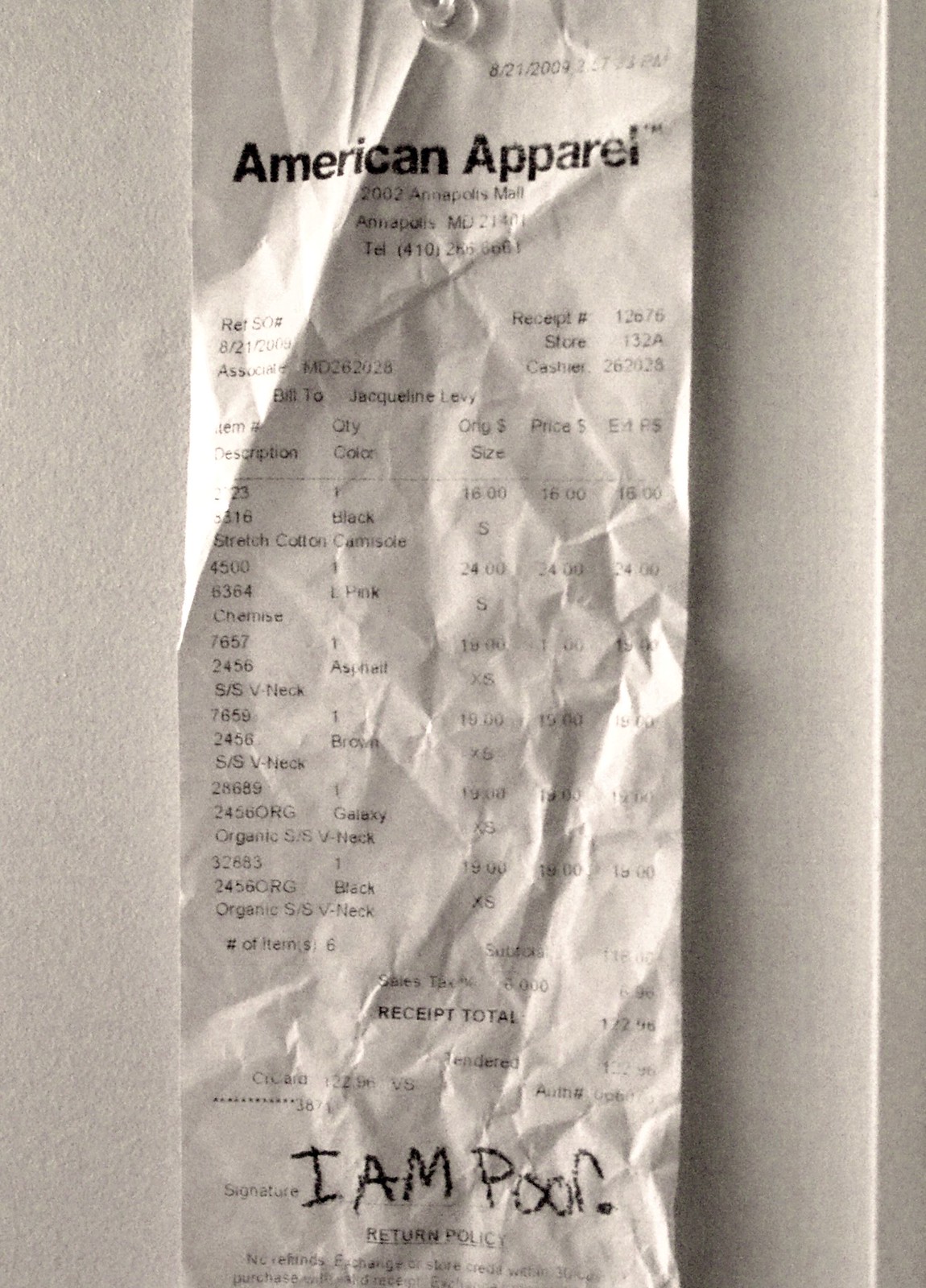In the image, a crinkled but straightened receipt from American Apparel is thumbtacked to a white wall using a clear push pin at the top. The receipt is from 8-21-2009 and lists items purchased at the 2002 Annapolis Mall location in Annapolis, Maryland. Although the lettering is somewhat faded due to previous crumpling, some details are discernible. The purchased items include various v-neck shirts such as a black camisole, a pink item, and a galaxy v-neck. The total amount of the purchase is $172.46 for six items. Notably, where the customer's signature would typically be, someone has humorously written "I am poor" in big block letters, likely with a colored pencil or crayon.